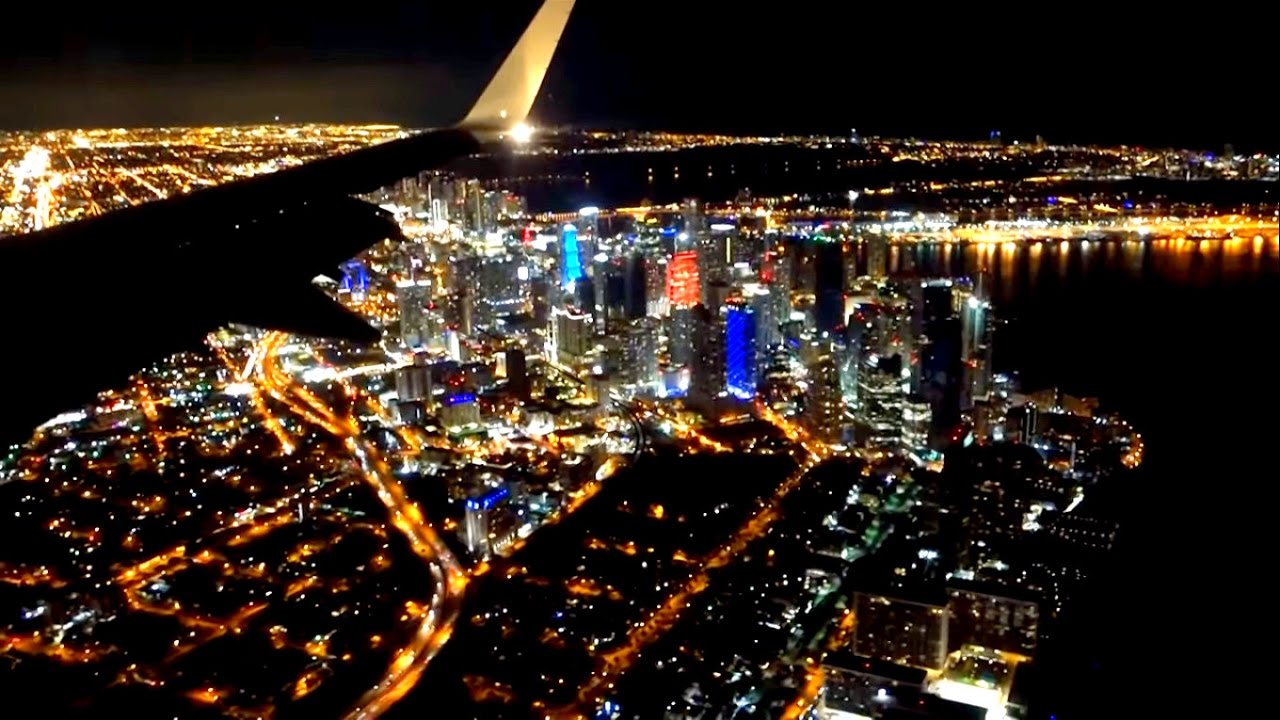This nighttime aerial photograph, taken from the window of a jetliner, captures the dazzling expanse of a large metropolitan city. The silhouette of the airplane's wing frames a sprawling urban landscape below, dominated by a cluster of towering skyscrapers in the city center. The city is crisscrossed by illuminated roads and highways, with the lights of countless vehicles creating a web of glowing arteries. The cityscape stretches out endlessly, with a vibrant mix of blue, orange, red, and green lights showcasing its dynamic character. In the foreground, a vast body of water, possibly a lake or river, reflects the city's lights, adding a shimmering quality to the scene. The water appears dark and blank except at its lit edges, emphasizing the bright, illuminated city that appears to extend for miles. Far in the distance, additional clusters of lights suggest neighboring cities or ports, although individual details are obscured by the brightness. This captivating image vividly portrays the bustling, illuminated heart of a heavily populated urban area at night.